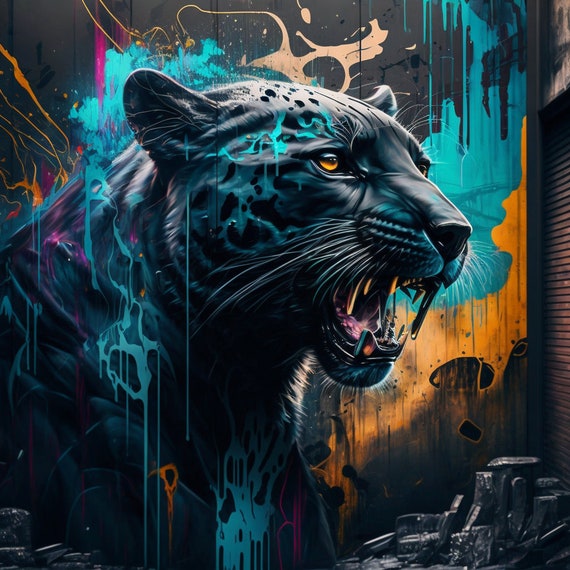In this striking piece of modern graffiti art, an enormous black feline head—most likely a panther—emerges from a vividly graffitied wall. The backdrop is a chaotic blend of teal, black, and yellow, interspersed with splashes of pink, turquoise, dark orange, peach, and beige. These vibrant colors form an abstract background that complements the striking central figure. The panther's face is adorned with teal lightning-like streaks, contrasting against its dark fur. Its mouth is open wide, revealing fangs that look like giant, metallic shards. The eyes of the beast are a captivating gold, and its small, proportionate ears add to its fierce appearance. Below this imposing figure is a textural element resembling rock or wood, catching and reflecting light. To the far right, the scene is bordered by a closed storefront with dark, slatted lines over a tan surface, adding an urban context to the artwork.